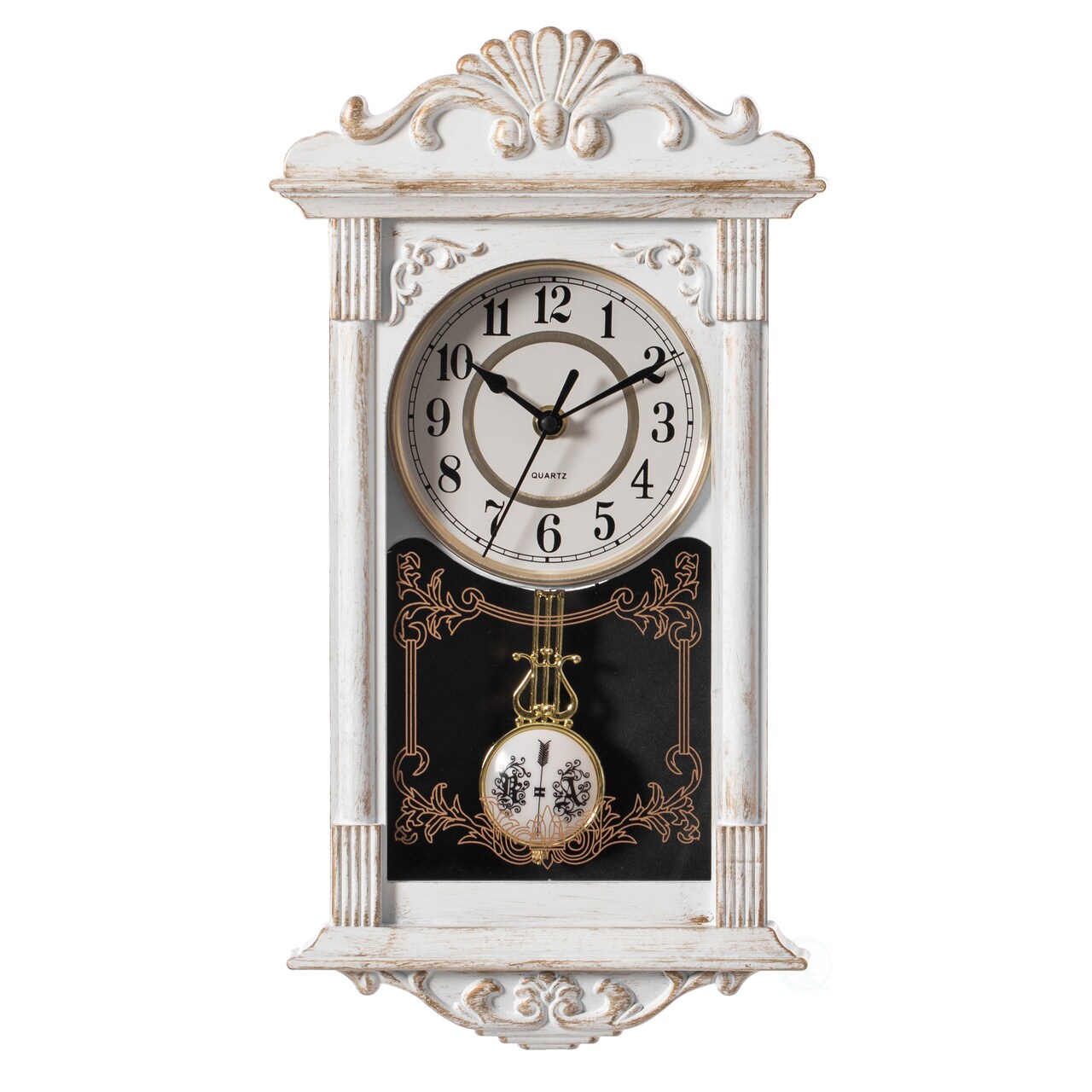This is a detailed photograph of an antique-looking wall-mounted clock, measuring approximately two feet high by one foot wide. The clock is housed in an ornate wooden frame, painted white and adorned with intricate scroll work at the top and bottom. The paint is worn in several places, revealing the underlying wood and giving it a rustic, aged appearance. 

The clock face is white with black numerals and hands, and it features a gold outline. The short hand points to 10, the long hand to 2, and the seconds hand to 7, indicating a time of around 10:10 and 34 seconds. Above the number six, the word "quartz" is inscribed in black.

Below the clock face hangs a sizable pendulum, which swings back and forth. The pendulum is mounted on a gold heart-shaped piece with decorative lines extending upward. The pendulum itself is white with gold accents and includes what appears to be an arrow motif, with the letters "A" on one side and an unclear letter on the other.

The background of the image is transparent, highlighting the clock's elaborate design. Despite its ornate and decorative features, the clock's age and the wear on its painted surface contribute to its vintage charm.